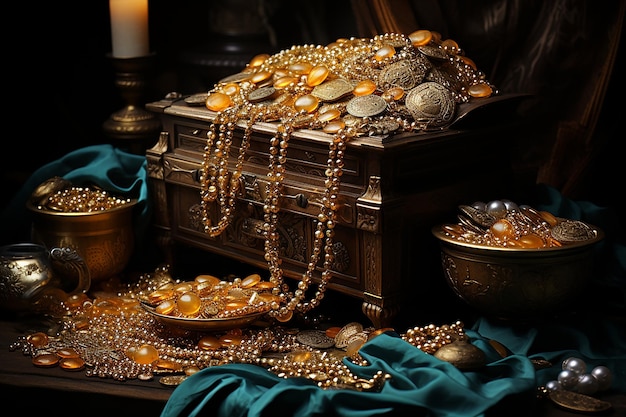The image depicts a highly detailed, AI-generated, 3D color illustration of a treasure chest scene set against a dark background, emphasizing the chest and its surroundings. The focal point is a large, dark wooden treasure chest with elaborate corner details, positioned at a slight angle with the front side facing the bottom left of the image. The chest is overflowing with an abundance of gold coins, strands of pearls, and various jewels, including necklaces and other ornate items. Flanking the chest are two bowls brimming with additional treasures, one on the left and one on the right, along with a shallow dish in front also filled with pearls and gold. Surrounding the setup, a turquoise silk scarf is draped elegantly in the bottom right corner and the top left next to the chest. A few gold nuggets and a small gold bucket can be seen on the side, hinting at the richness of the collection. The scene is completed with a pillar candle, partially visible on the top left, and several silver balls scattered in the bottom right corner. This intricate and visually captivating arrangement evokes the impression of a pirate’s bountiful treasure hoard displayed on a table.